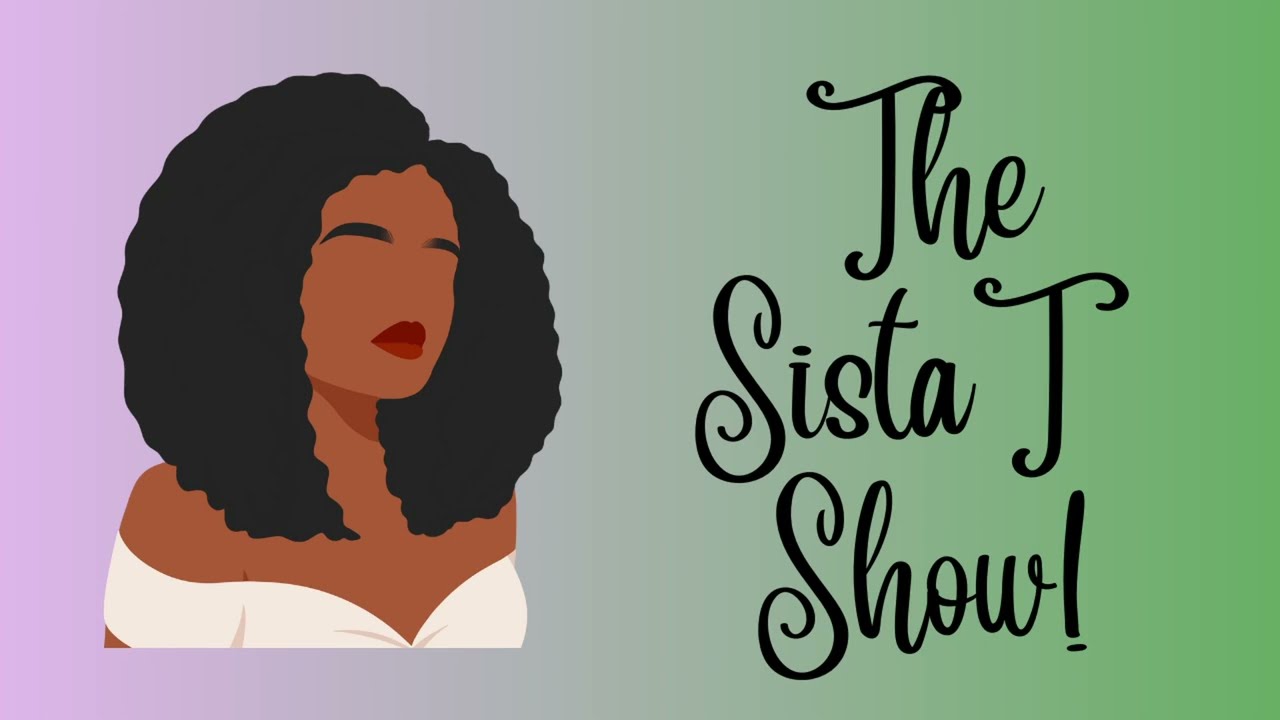The image features a banner likely for a podcast or live stream titled "The Sista T Show." The title, written in black, whimsical cursive text with an exclamation mark at the end, is positioned on the right side. On the left side, there is a cartoon-style illustration of an African-American woman with thick curly hair flowing down to her shoulders. The woman, depicted with dark eyebrows, big red lips, and without a nose or eyes, wears a white top with straps on both sides, leaving her shoulders bare. The background exhibits a gradient blend from pastel purple on the left to pastel green on the right, creating a vibrant and visually appealing backdrop. The overall style of the illustration is reminiscent of the corporate Memphis style, emphasizing simplicity and minimal defining features.